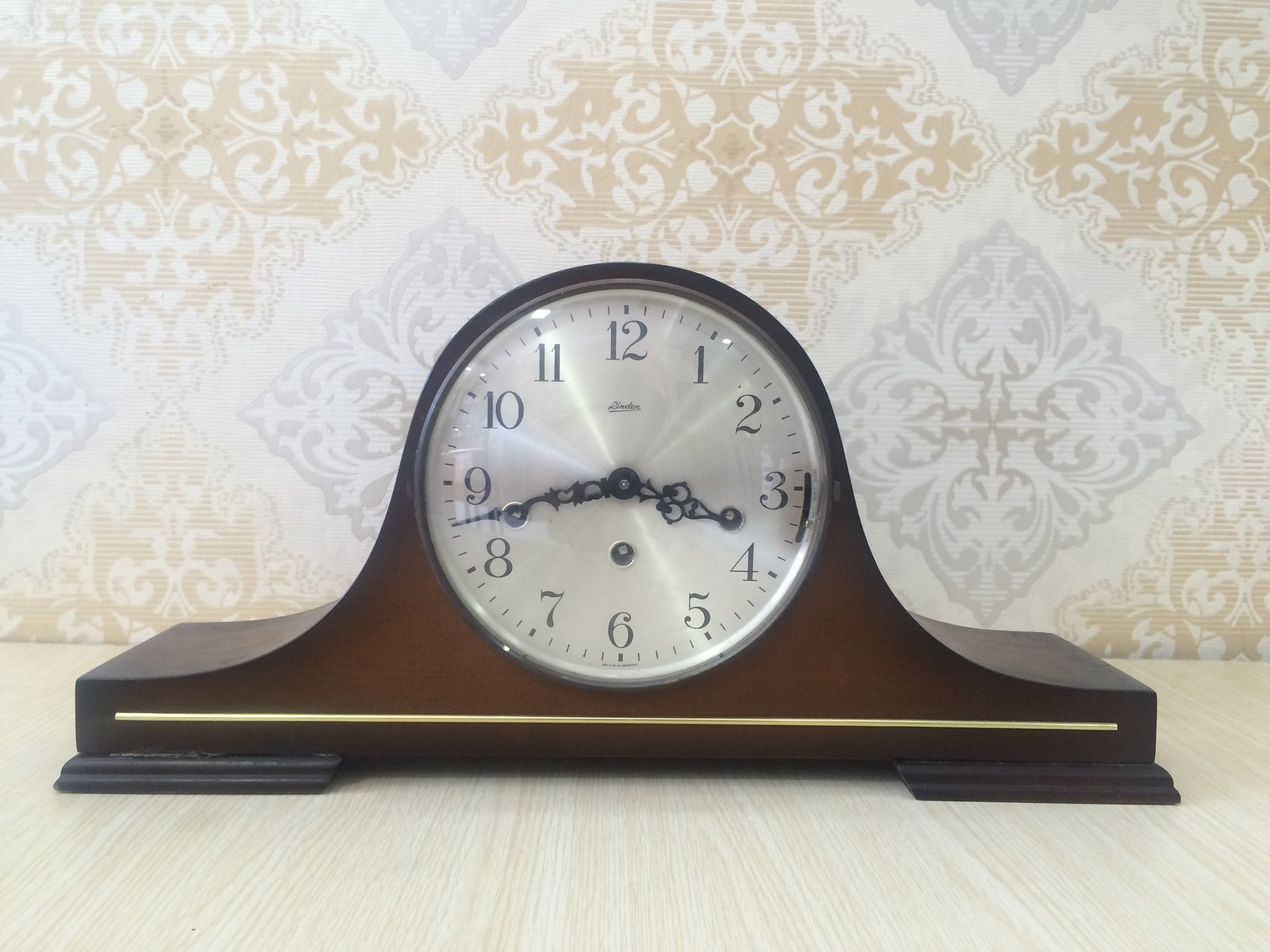This photograph showcases a beautifully crafted chocolate-brown wooden clock, elegantly displayed on a light-colored surface that reveals the detailed wood grain. The clock is adorned with a gold line beneath its silvery-white, round face. Encased in glass, the face features intricate, floral-patterned black hands and clearly visible black numbers. The light reflecting off the glass adds a touch of elegance to the timepiece. In the background, there is a charming wallpaper with a floral pattern in shades of tan, gray, and white, adding a vintage and cozy ambiance to the scene.